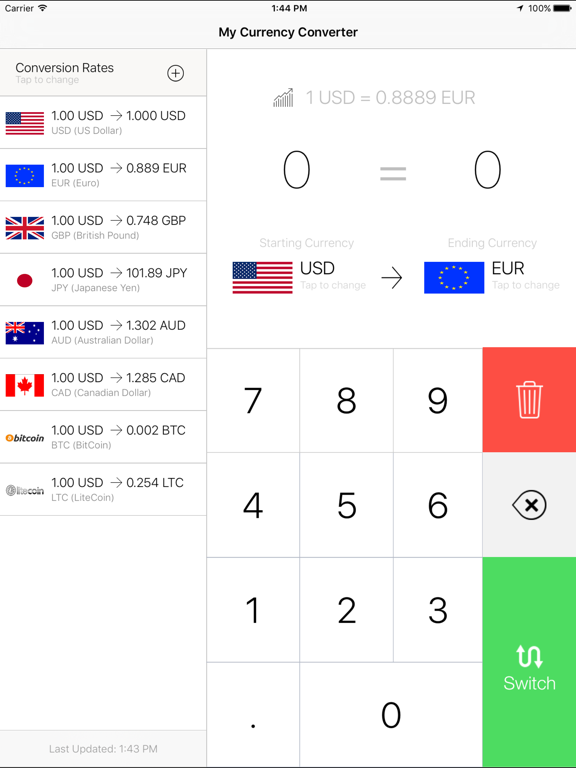In this screenshot, against a solid white background in the upper left corner, there is black text displaying the carrier name, accompanied by a Wi-Fi icon. At the center top, the time is shown as 1:44 p.m. in bold black text next to the title "My Currency Converter." In the upper right corner, the battery status is displayed as 100%.

Starting from the left, there is vertically aligned text that reads "Carrier," "Conversion Rates," and below that, a series of currency conversions. The first conversion shows the U.S. flag with exchange rates from $1 USD to several denominations, including increments up to $1,000 USD. Directly below, it indicates that $1 USD equals 0.889 EUR. 

Following this, there is a British flag illustrating the exchange rate, where $1 USD converts to 0.748 GBP. The next line shows that $1 USD equals 1,089 JPY, marked by the Japanese yen symbol. The final conversion details are accompanied by an Australian flag, indicating that $1 USD equals 1.302 Australian dollars.